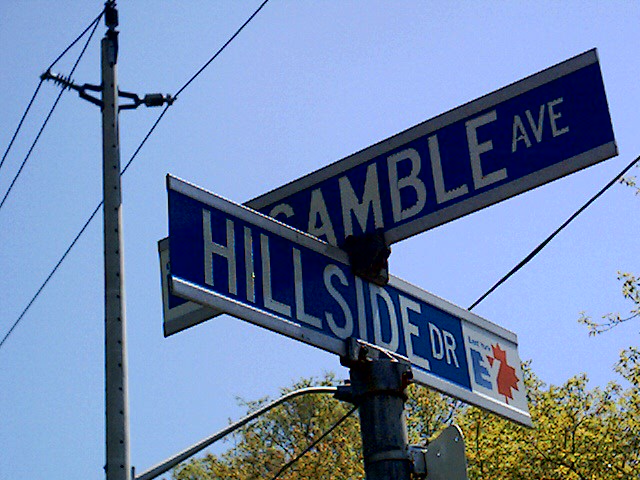A photo captures a crisp, clear day, showcasing a blue sky above a street intersection marked by a distinct street sign. The sign indicates the crossing of Hillshire Drive and Gamble Avenue, possibly situated in Canada, as suggested by a logo on the right side of the Hillshire Drive sign, resembling a maple leaf, an iconic symbol associated with Canadian imagery. Nestled under a network of power and telephone lines, the street signs are mounted on a sturdy metal pole, reinforced with silver brackets at the top and bottom. A backdrop of lush green trees adds a touch of nature to the scene, beautifully complementing the industrial elements of the power lines and street infrastructure.